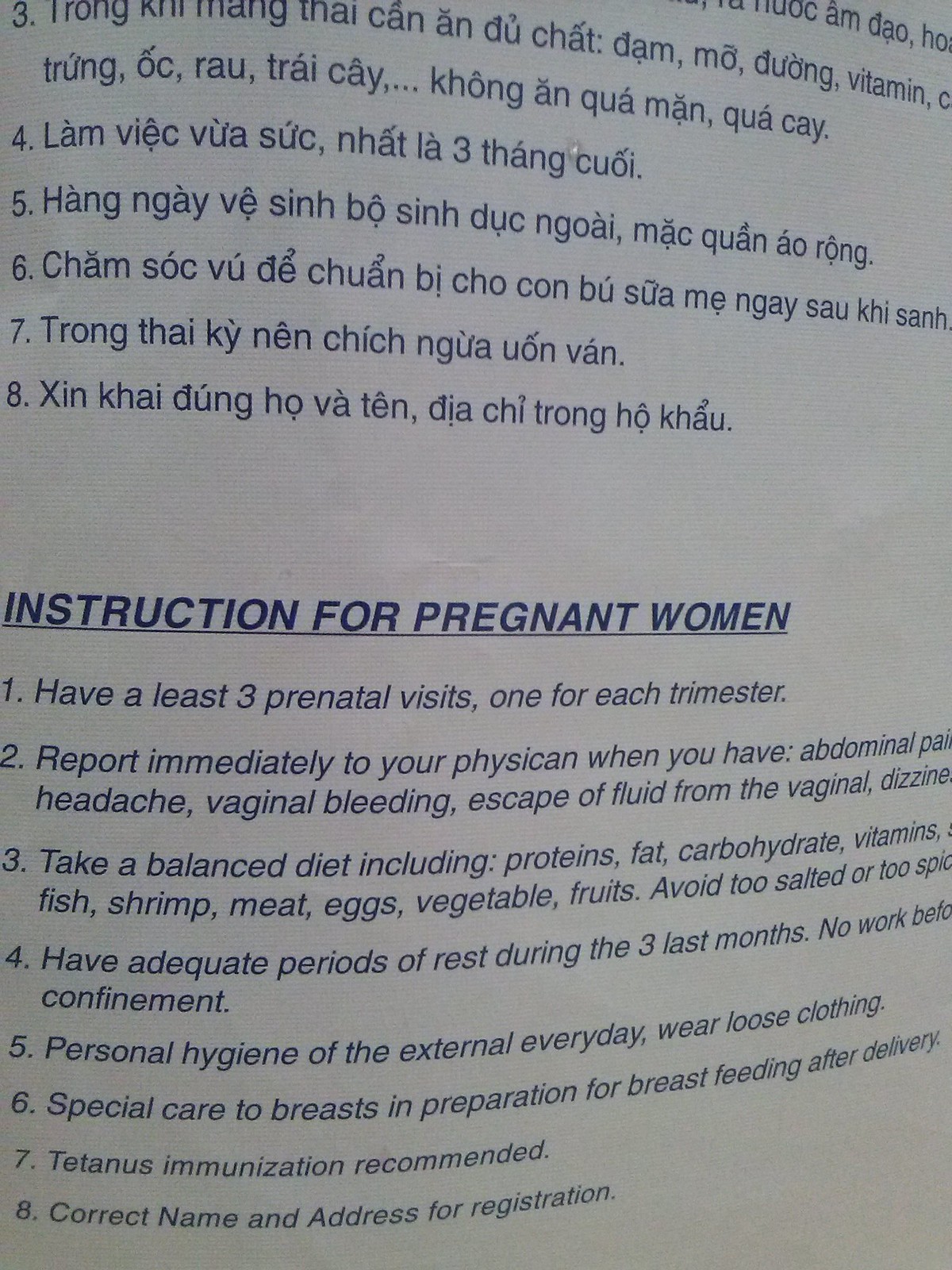The image displays a slightly twisted piece of paper with a bent corner, featuring text from what seems to be a magazine or book. The top section of the page is filled with text in Vietnamese, while the lower portion has an English translation in italicized, sans-serif black font. The English section is titled "Instructions for Pregnant Women" in bold and underlined. Below the title, there are eight detailed guidelines for expecting mothers:

1. Have at least three prenatal visits, one for each trimester.
2. Report immediately to your physician when you experience abdominal pain, headache, vaginal bleeding, escape of fluid, or dizziness.
3. Maintain a balanced diet including proteins, fat, carbohydrates, vitamins, fish, shrimp, meat, eggs, vegetables, and fruits. Avoid overly salted or spicy foods.
4. Ensure adequate rest periods during the last three months; abstain from work before confinement.
5. Practice daily personal hygiene and wear loose clothing.
6. Give special care to the breasts in preparation for breastfeeding after delivery.
7. Tetanus immunization is recommended.
8. Ensure your correct name and address are registered.

The instructions provide comprehensive prenatal care advice, emphasizing balanced nutrition, regular medical check-ups, personal hygiene, and rest.